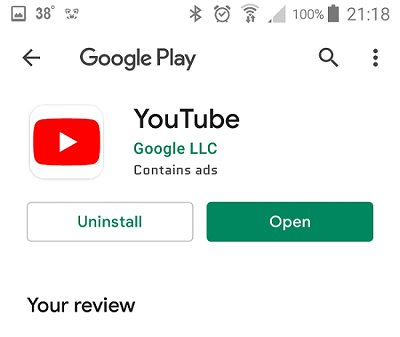The image appears to be a partial screenshot taken from a smartphone. The screenshot captures roughly half of the phone's display. 

**In the top-left corner:**
- A small picture icon is visible.
- Next to the picture icon, the temperature is displayed as "38°". 
- An unidentified icon is situated adjacently.

**Centered at the top of the image:**
- There are several key status icons arranged in a row: 
  - A Bluetooth icon.
  - A clock icon.
  - A Wi-Fi icon.
  - A signal strength icon, which shows about a quarter of full signal.

**To the far right, at the top:**
- The battery icon appears fully charged.
- The time is displayed in military format as "21:18".

**Underneath the status bar:**
- To the left, an arrow pointing left is visible.
- "Google Play" is displayed.
- To the right, there's a magnifying glass icon followed by three dots.

**Dominating the center-lower part of the image:**
- A large box with rounded edges and a white background houses the YouTube logo. 
  - The YouTube icon appears prominently.
  - Next to the icon, "YouTube" is shown, aligned and centered.
  - Below "YouTube," "Google LLC" is written in green font, with "contains ads" beneath it.

**At the bottom of the image:**
- Two prominent buttons labeled "Install" and "Open" are presented, with the "Open" button featuring a green background.
- Underneath these buttons, "Your review" is mentioned on the left side.

This detailed description highlights the key elements visible within the partial screenshot from the smartphone, successfully conveying the contents and layout of the image.